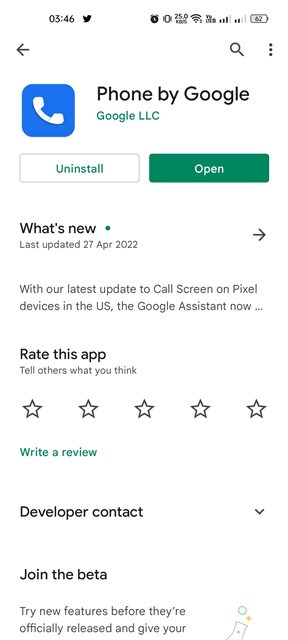This screenshot showcases the Google Phone application interface. Dominating the top section is a blue phone icon. Directly beneath, two functional buttons are displayed: an "Uninstall" button and an "Open" button, the latter is highlighted in green with the word "Open" in bold white text. 

Below these buttons, the section titled "What's new" reveals that the app was last updated on April 27, 2022. An arrow pointing to the right leads to further details, which mention enhancements to the Call Screen feature on Pixel devices in the U.S., noting that the Google Assistant has received updates.

Further down, users are invited to "Rate this app" and share their thoughts. This section features five stars outlined in black and filled in white, alongside the prompt "Write a review."

At the bottom of the screenshot, two additional options are presented: "Developer contact," which can be expanded by clicking a downward-pointing arrowhead, and "Join the beta," inviting users to try new features before their official release. The accompanying subtext provides more insight into these beta opportunities.